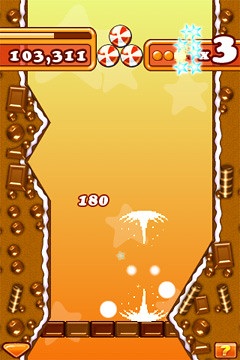The image is a screenshot from a mobile candy-themed game featuring a gingerbread house design. The background displays a light brown chocolate outline with a white edge on both sides, giving a gingerbread house effect. At the top left corner, inside an orange rectangle with a red trim, there is a partially filled power bar and a total score of 103,311 in white numbers. Centered at the top are three red-and-white peppermint candies, suggesting a game's objective related to candies. The top right features blue stars and an indicator displaying "x3," possibly a multiplier or inventory. The image also showcases various candies and chocolate pieces scattered throughout. Two splash marks or popping bursts are visible in the center, adding dynamic elements. Throughout the image, various chocolate elements, including little round bars, square chocolate pieces, and something resembling a Rolo in the center, further emphasize the candy theme.